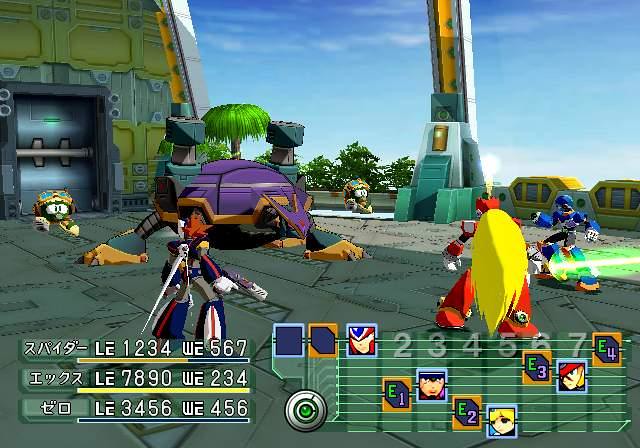This image captures an action-packed moment from a Japanese video game, likely from the Mega Man series, featuring a detailed battle scene set against a vibrant blue sky with clouds. The background showcases a large yellow structure, resembling a headquarters or garage, near the top left of the image. The battlefield is divided, with the "good guys" positioned at the bottom and the "enemies" at the top.

On the bottom right, we see a character with long blonde hair, dressed in a red suit and wielding a green sword. Next to him is a figure reminiscent of Mega Man, clad in a blue outfit and carrying a weapon. There’s also another character on the bottom left, sporting brown hair and a blue suit, armed with a laser gun. The bottom features a grid displaying character faces and their health information, accompanied by Japanese writing and numbers.

Prominently positioned in the battle is a large purple creature, resembling a turtle, protecting the yellow structure in the background. This creature is flanked by enemy characters that look like bombs with faces. The overall scene is incredibly dynamic, emphasizing the vibrant colors and detailed graphics that bring the confrontation to life.